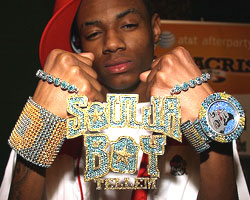The image features a close-up of the rapper, Soulja Boy (spelled S-O-U-L-J-A B-O-Y). He is captured from the upper chest to just above his eyebrows and is facing the camera. The background is dark, with an orange sign bearing the AT&T logo visible on the right side. Soulja Boy is holding up a large, diamond-encrusted pendant. The pendant spells out "Soulja Boy" in teal and gold letters, with "tell 'em" emblazoned beneath in gold diamonds.

Soulja Boy wears a red baseball cap tilted over his right ear and a white shirt with a red stripe. His fists are raised to his cheeks, and across them hangs the thick chain of the pendant, adorned with teal diamonds. On his left wrist, he sports an oversized gold and blue diamond watch, and on his right wrist, a wide bangle that extends from his wrist to mid-forearm, featuring similar blue and gold jewels. His expression remains neutral as he showcases his extravagant accessories.